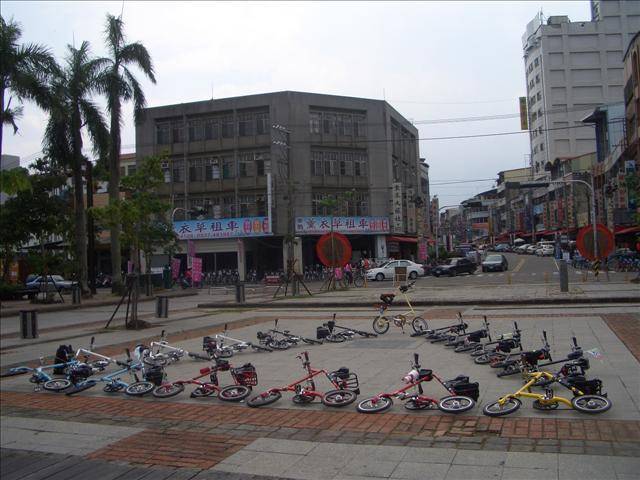This photo was taken outdoors in an Asian city, evidenced by the writing on some of the signs visible in the image. The scene features a busy street with an intersection on the right side, displaying several cars merging onto the road. The perimeter of the street is lined with buildings, including a multi-story structure with Asian characters on a sign. Alongside the city, there are palm trees visible to the left. Central to the image is a town square that includes a courtyard with a stone-tiled walkway. In the middle of the square, a notable triangular pattern of bicycles, varying in colors such as yellow, red, white, and blue, lies on the ground. These bikes appear to be e-bikes, perhaps available for rental. Interestingly, one bike at the tip of the triangle stands upright, contrasting with the others.